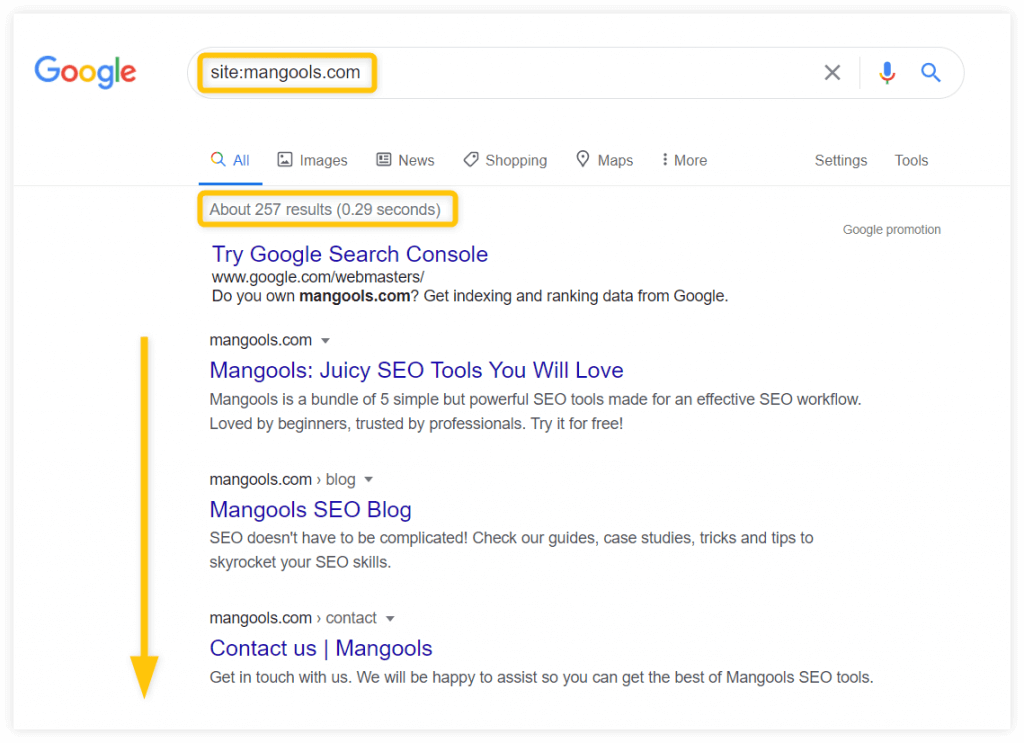In the upper-left corner of the image, the word "Google" is prominently displayed. To the right of this, within a yellow highlighted box, is the text "site: mangools.com" typed into the search bar. Directly below the search bar, the word "All" is underlined in blue, indicating it's the active search category. Adjacent to it are other categories such as "Images," "News," "Shopping," "Maps," "More," "Settings," and "Tools," all outlined in a yellow box. Within this yellow box, it also mentions "About 257 results (0.29 seconds)" indicating the number of results and the speed of the search.

A long yellow arrow on the left side of this section points downward, drawing attention to clickable options that are displayed in blue. 

The first result is prominently titled "Try Google Search Console."

- The second result reads "Mangools," followed by a subtitle "Juicy SEO Tools You Will Love."
- The third result is labeled "Mangools SEO Blog."
- The fourth result is simply "mangools.com."

Underneath these is a blue link that says "Contact Us," followed by a vertical line and another link titled "Mangools." The text beneath this link reads: "Get in touch with us. We will be happy to assist you so you can get the best of Mangools SEO tools."